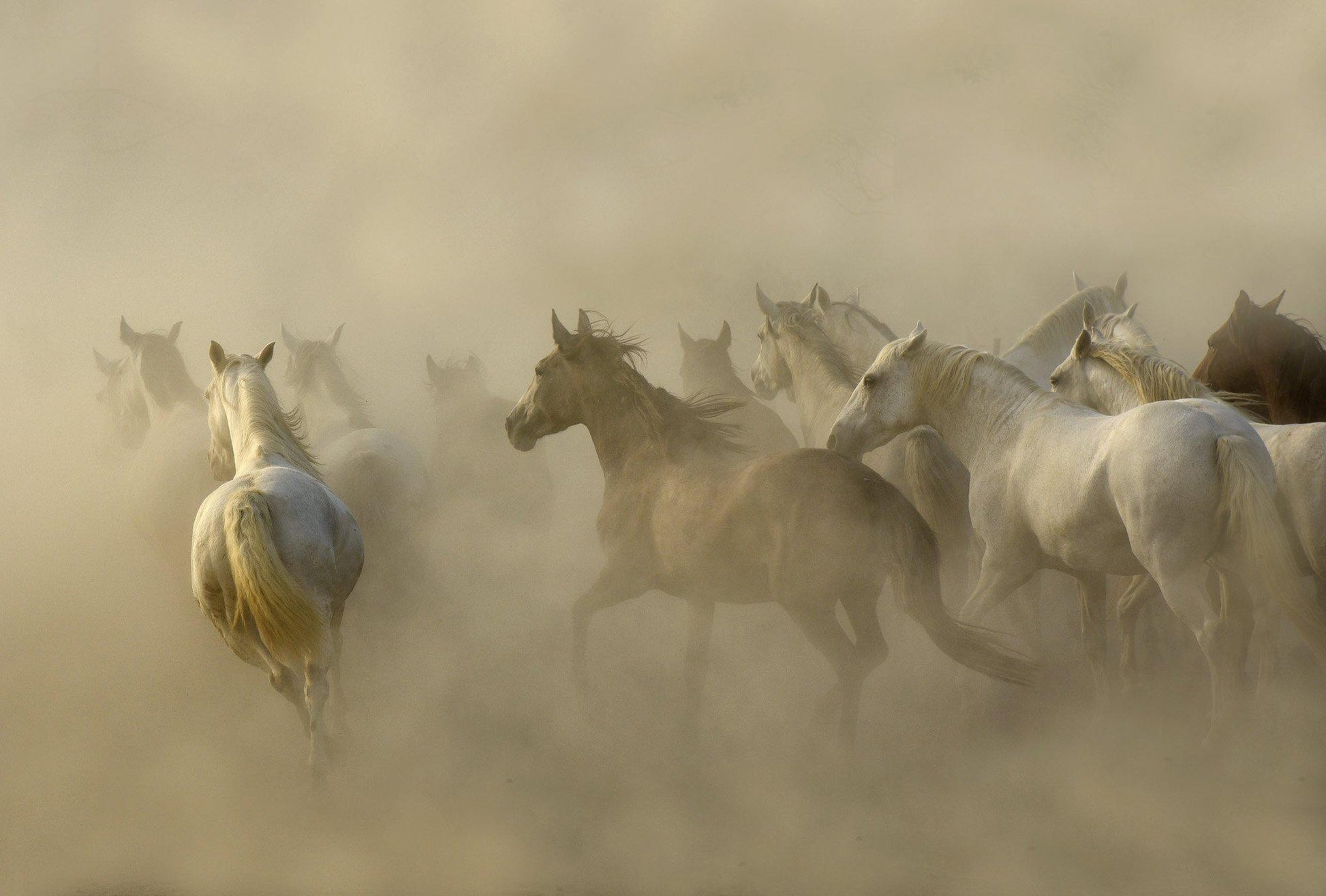The image is a stunning piece of art, possibly a highly intricate digital painting or drawing rendered with such precision that it almost resembles a photograph. It depicts over a dozen horses in a dynamic stampede away from the viewer. The majority of the horses are white, with a few highlighted in various shades of brown, including a striking dark mahogany and a lighter brown. The horses appear to be in a state of exhilarated frenzy, their manes flying wildly as they kick up clouds of dust, which almost blend them into a foggy, gray background. The scene is so enveloped in dust and mist that the surrounding landscape is obscured, creating a dramatic effect of motion and energy. Despite the lack of an artist signature, the beauty and detail of the piece make it a captivating display of wild horses galloping through a haze, their forms fading into the plumes of dust they've created.